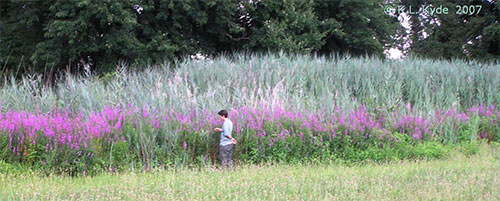In this detailed outdoor landscape scene, likely a painting, the focal point is a lone figure standing in a vibrant field. The person's gender is ambiguous, possibly a man or woman, with either brown or dark hair, dressed in a white shirt and brown or purplish pants. They stand contemplating a line of tall, magenta-pink flowers that stretch across the foreground. Surrounding this figure, the scene is rich with textures and layers: a mixed carpet of yellow and green grass, about a foot or two high, lies at the bottom, while behind the flowers stands a wall of towering, light green grasses, nearly double the person's height. As the eye moves further back, there's a dense forest of trees that frames the scene. The sky above is scattered with clouds, and a gentle light filters through on the right side. The overall effect is a serene, yet vivid portrayal of a person deeply engaged with their natural surroundings.